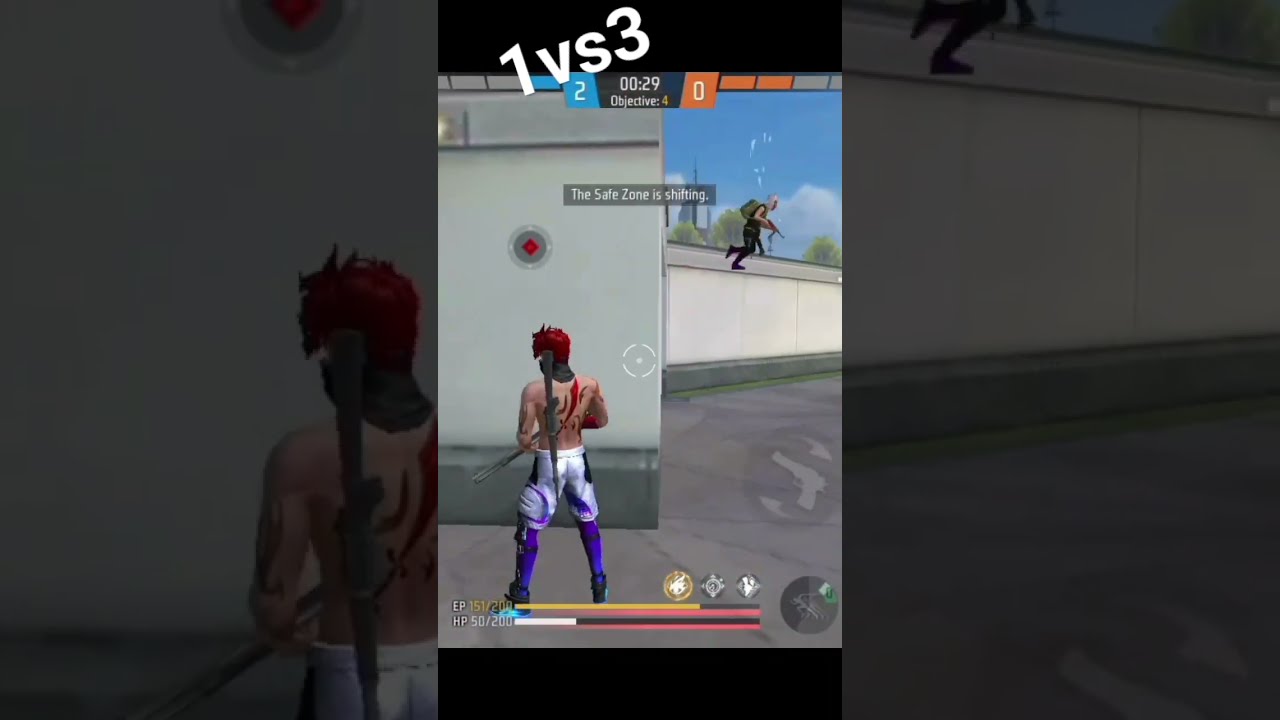The image is divided into three vertical sections. The first and third sections are darkened close-ups of the central section, where the focus is on a screenshot from a third-person shooting video game. The central section depicts two characters. The main character, who occupies the left side of this section, has red hair, no shirt, white skin, a back tattoo, and white pants with purple elements. He is holding a gun and facing away from the viewer. On the right, another character is in mid-air, seemingly jumping over a white wall, also holding a gun and dressed in a black outfit with a belt. The background consists of gray ground and a building between the characters. At the top of the central section, white text reads "1 vs 3." Further down, it displays a score of "2-0," a timer at "29 seconds," and the text "objective 4." At the center, more white text announces that "the safe zone is shifting." The bottom edge of the image includes various icons and statistics, possibly indicating health and other game metrics.